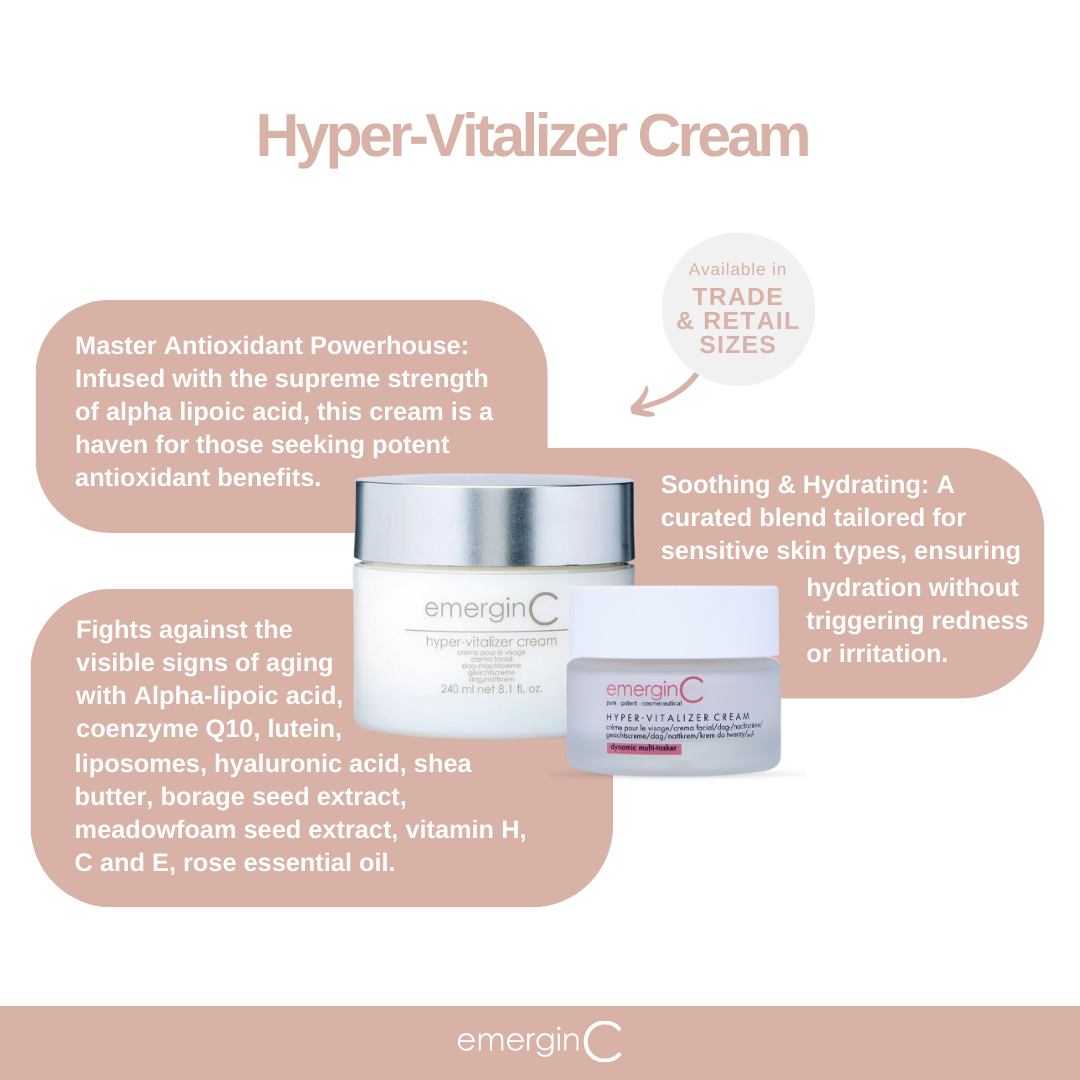This advertisement for Emergen-C hypervitalizer cream is intricately detailed and elegantly designed. Set against a rose beige background with white accents, it prominently features the sophisticated skincare product, emphasizing its powerful antioxidant benefits. At the very top, "Hypervitalizer Cream" is highlighted, drawing attention to its potent formulation.

The ad showcases two jars of Emergen-C: one with a silver lid and white bottom, and the other with a white lid and clear bottom, both artfully placed atop a trio of rounded-corner rectangles. A circular callout indicates the product's availability in both trade and retail sizes.

Central to the ad's messaging is the cream's description as a "Master Antioxidant Powerhouse" infused with alpha-lipoic acid, coenzyme Q10, lutein, liposomes, hyaluronic acid, shea butter, borage seed extract, meadowfoam seed extract, and vitamins H, C, and E, complemented by rose essential oil. This formulation is specifically curated for sensitive skin, ensuring hydration without causing redness, and effectively fighting visible signs of aging.

The bottom of the ad features a band with the "Emergen-C" brand name in large, white type, tying together the image's clean and professional aesthetic.